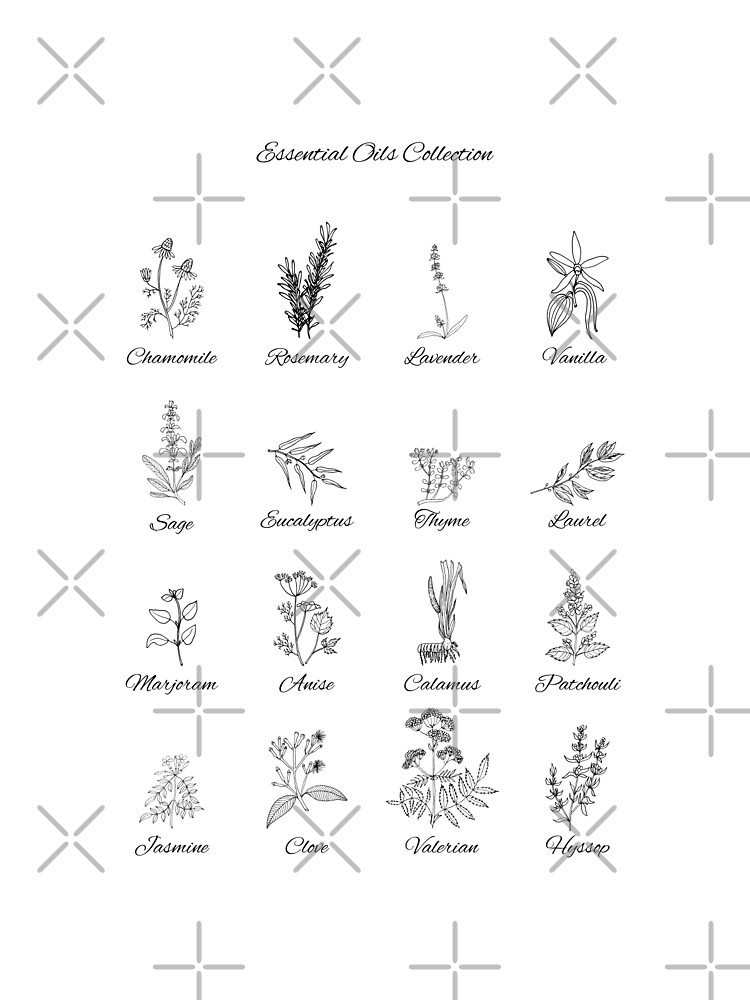This image, titled "Essential Oils Collection" in black cursive text at the top, features a grid of small, detailed black-and-white drawings of various plants against a white background. The layout consists of four rows with four illustrations each, showcasing individual plant parts such as stems or leaves. The annotated plants, from left to right and top to bottom, are Chamomile, Rosemary, Lavender, Vanilla, Sage, Eucalyptus, Thyme, Laurel, Marjoram, Anise, Calamus, Patchouli, Jasmine, Clove, Valerian, and Hyssop. The clarity of the image is compromised by pervasive watermarks, consisting of X and cross shapes in gray, which obscure some of the text and drawings. Despite the watermarks, the intricate line art of each plant is discernible, drawn meticulously as if with a fine marker or pen.